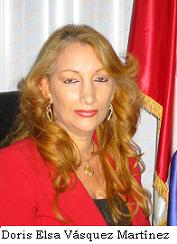This indoor photograph features Doris Elsa Vasquez Martinez, as indicated by the text beneath the image. Doris is seated in a black chair and set against a backdrop that includes a white curtain. On the right side of the image, there's a flag, likely of official significance, displaying red, white, and blue colors with yellow fringe along its bottom edge, attached to a flagpole. Doris has wavy, blondish, or possibly reddish-blonde hair that is styled neatly. Her eyebrows are manicured, and she wears eyeliner and red lipstick. Her attire includes a red dress jacket over a black camisole or t-shirt, along with dangling earrings and a necklace. Her expression is a subtle smile, appearing almost as a smirk, and the photo captures her from the chest up.